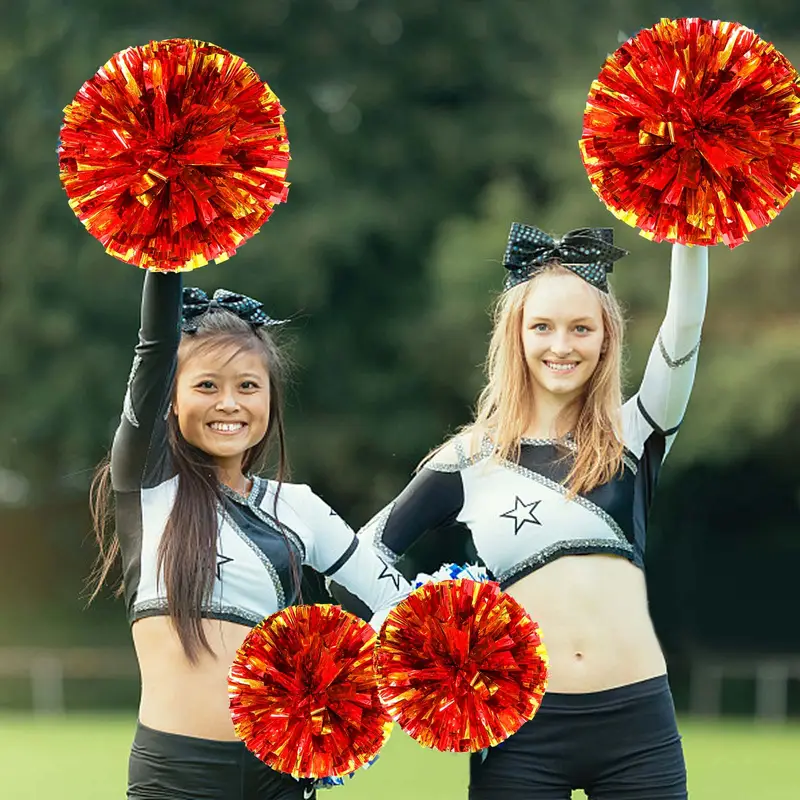In this image, two young cheerleaders are posing outdoors in front of a large tree and a possibly white, blurry fence in the background. Both are dressed in identical black and white long-sleeve crop tops that reveal their midriffs and feature a diagonal design with a star over the chest, paired with black bottoms. They are holding large, red pom-poms flecked with hints of yellow or orange; one pom-pom is raised while the other rests near their waists.

The cheerleader on the left appears to be of Asian descent, with long, brown hair styled in a half-ponytail, secured by a black bow with white checkered or green sequined designs. She has a big smile on her face. Her counterpart on the right is slightly taller, with pale skin, blonde hair tied back with a similar ribbon, and blue eyes. She, too, is smiling brightly. Both cheerleaders display a joyful camaraderie, highlighting their spirited enthusiasm in matching attire and coordinated poses.